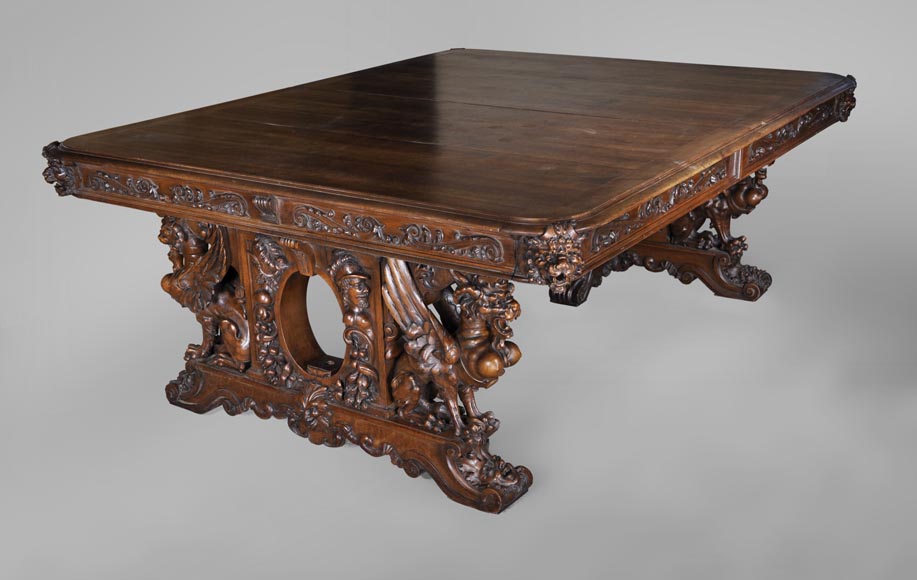This image features a horizontally aligned rectangular photograph of a highly ornate wooden table set against a plain, medium gray background blended with some white, giving it a cloudy or mottled appearance. The table, an older and dark-stained piece, dominates the composition. Its glossy top showcases a blend of lighter and darker wood grains, creating a smooth, visually rich surface.

The sides of the table are adorned with intricate carvings, including swirling patterns, griffins, and perhaps even figures of animals and people, adding to its richness. The table's legs are equally elaborate, with each pair of legs thick and wide, appearing as though carved from single pieces of wood. These legs feature circular cutouts in their centers and are decorated with intricate designs and imagery, possibly including wings, round knobs, and mythical heads like those of elephants or dragons, with mouths open. The legs are curved, contributing to the table's grand and elaborate aesthetic. The photograph, devoid of any other elements such as text, shadows, or additional colors, focuses entirely on the ornate craftsmanship of the table, making it appear almost as if it were floating in this soft, nondescript background, reminiscent of a catalog image from a high-end auction house.